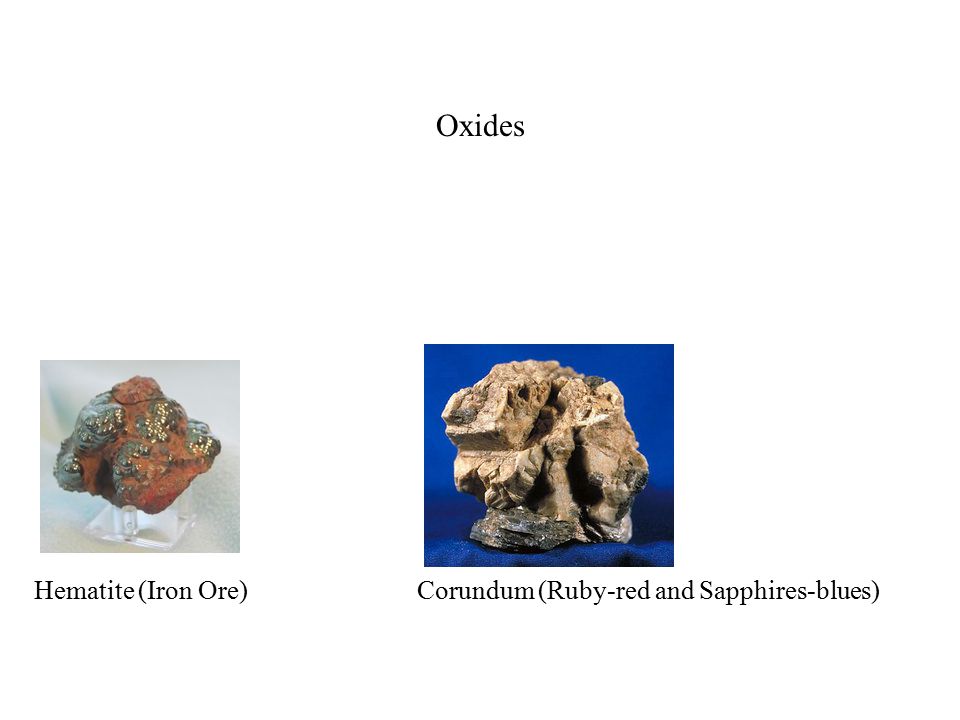The image features two photographs of different types of stones under the heading "Oxides" at the top against a white background. The left photograph shows a small, reddish stone with gold and gray flecks, placed on a plastic stand, with "Hematite (Iron Ore)" labeled underneath. The stone appears to be smaller than an apple and is presented against a white background. The right photograph displays a tannish stone with various grooves and divots, set against a blue background, and labeled "Corundum (Ruby Red and Sapphire Blue)."